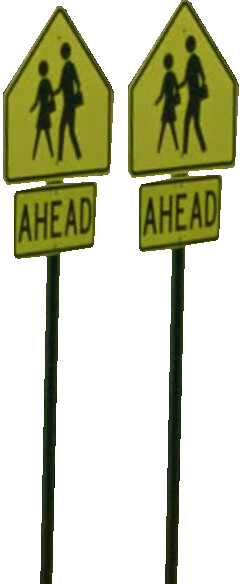The image features two nearly identical street signs designed to alert drivers to upcoming pedestrian crossings. Each sign has a distinctive design where the top portion resembles a triangular house and prominently displays the silhouette of two individuals walking. Below this, a small rectangular section bears the word "AHEAD" in bold, capital letters (A-H-E-A-D). The signs are mounted on a sturdy blue metal pole, which is embedded into the ground, typically in either dirt or concrete. These signs serve as crucial indicators for motorists to anticipate pedestrians crossing the street ahead.